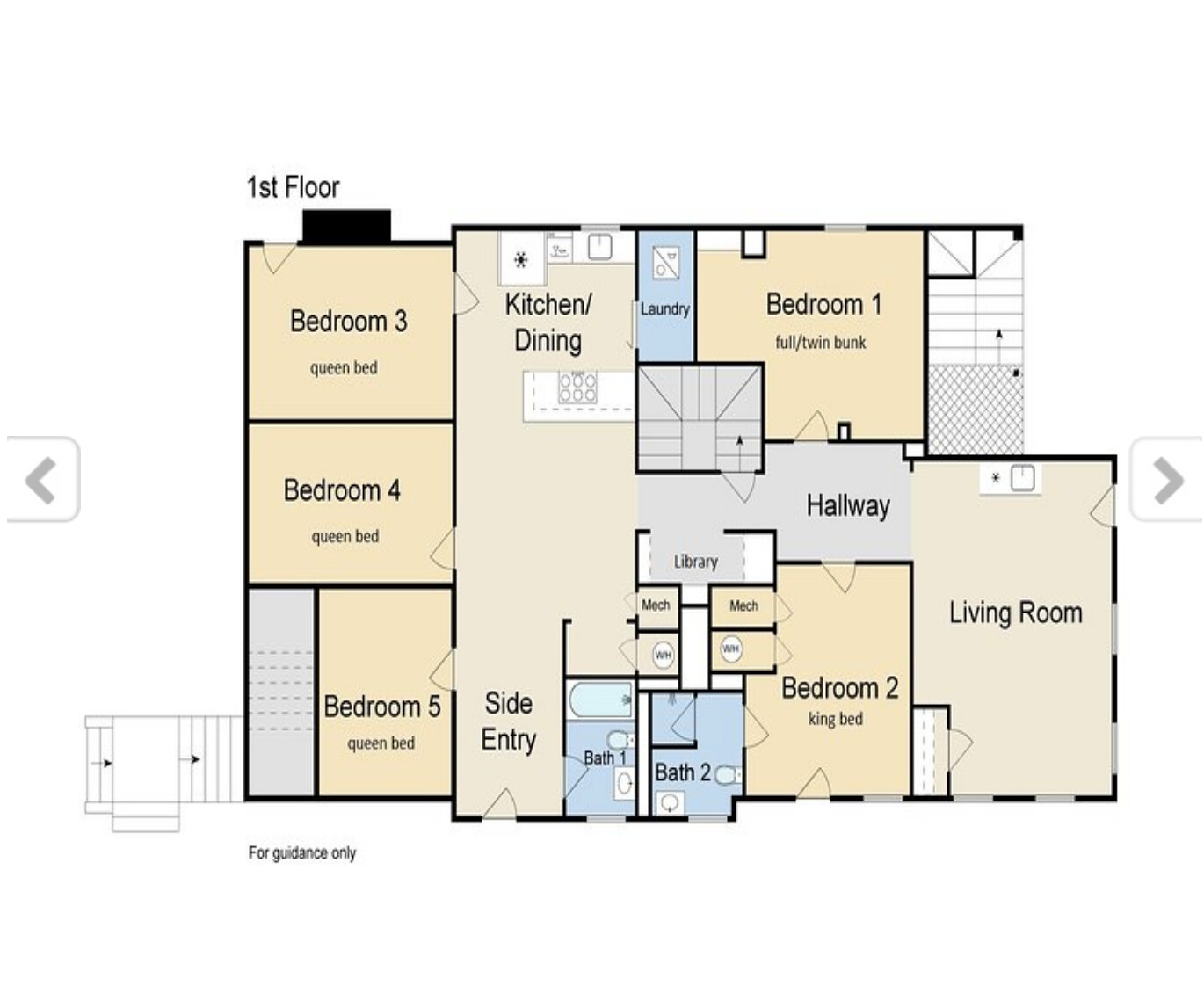**Detailed Layout Description for House Plan:**

From the left of the image, we see Bedroom 4 and Bedroom 5, each furnished with a queen bed. Moving towards the center, the kitchen and dining area are prominently featured alongside the laundry room. On the right side of the layout, Bedroom 1 is situated. Between Bedroom 1 and the central area, a hallway leads to a full twin bunk bed. The layout also includes a living room space. Additionally, there is a side entry, a library, two bathrooms (marked as Bathroom 1 and Bathroom 2), and another full twin bunk area. The background is white, with the note "For guidance only" at the bottom, indicating that this is a preliminary or conceptual plan.

**Note:** The layout information is for guidance purposes only and may not represent the final or actual arrangement.